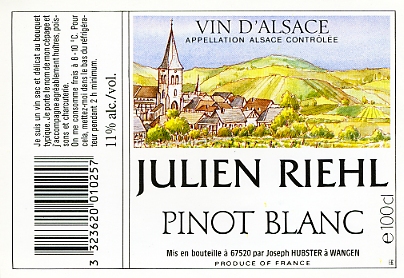The image captures a detailed label of a wine bottle called "Julien Riel Pinot Blanc," a product of France. The label, laid flat against a white background likely of a computer screen, features divided sections. On its left side, there's a vertically aligned panel with French text, a barcode, and the notation "11% alcohol by volume." The prominent right panel is square-shaped and displays an intricate, almost watercolor-like illustration of a charming village scene. This scene includes a prominent church steeple surrounded by smaller homes and green hills. At the top, "Vin d'Alsace" and "Appellation Alsace Contrôlée" are inscribed in black letters. Central to the label, "Julien Riel Pinot Blanc" is boldly indicated, affirming its French origin. Additionally, the label contains regulatory and product information, suggesting care in handling and consumption.